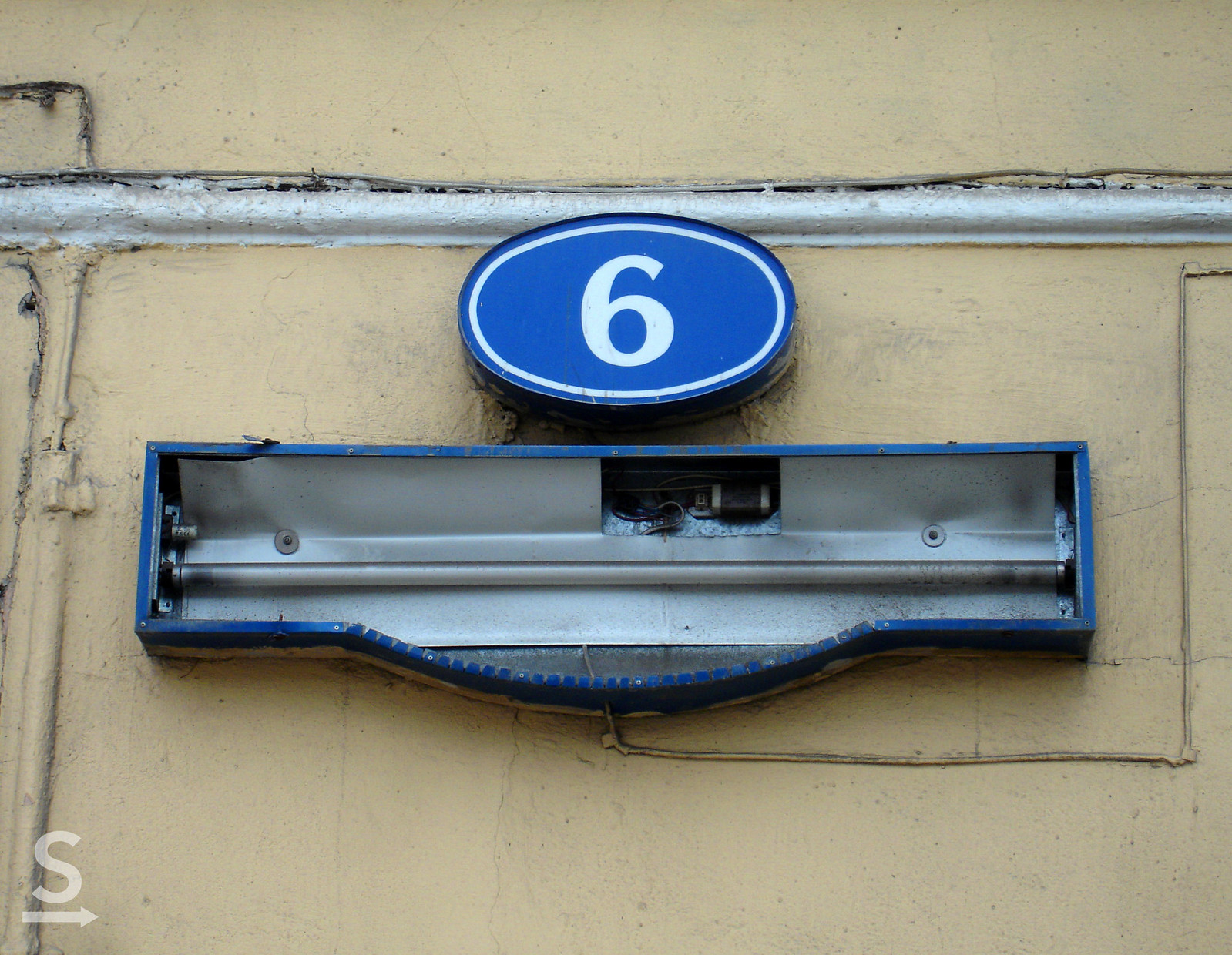In this outdoor color photograph, a tan concrete wall is partially covered with metal electrical conduits and white-painted molding. At the center of the image, a prominent blue oval sign with a white border features the number six. This sign likely has illumination capabilities, suggested by its design. Below this sign is a broken, upside-down, arched rectangular sign akin to the Sesame Street sign, also blue. The lens cover is missing, revealing its inner workings: a single horizontal fluorescent tube that appears burnt out, with another tube missing altogether. Electrical wires, clamped and painted tan to blend with the wall, run from the sign to the right. Additionally, there is a horizontal white line across the image near the top of the photograph, potentially a cable raceway or molding. In the bottom left corner of the image is a watermark featuring a white letter 'S' with an arrow pointing to the right.